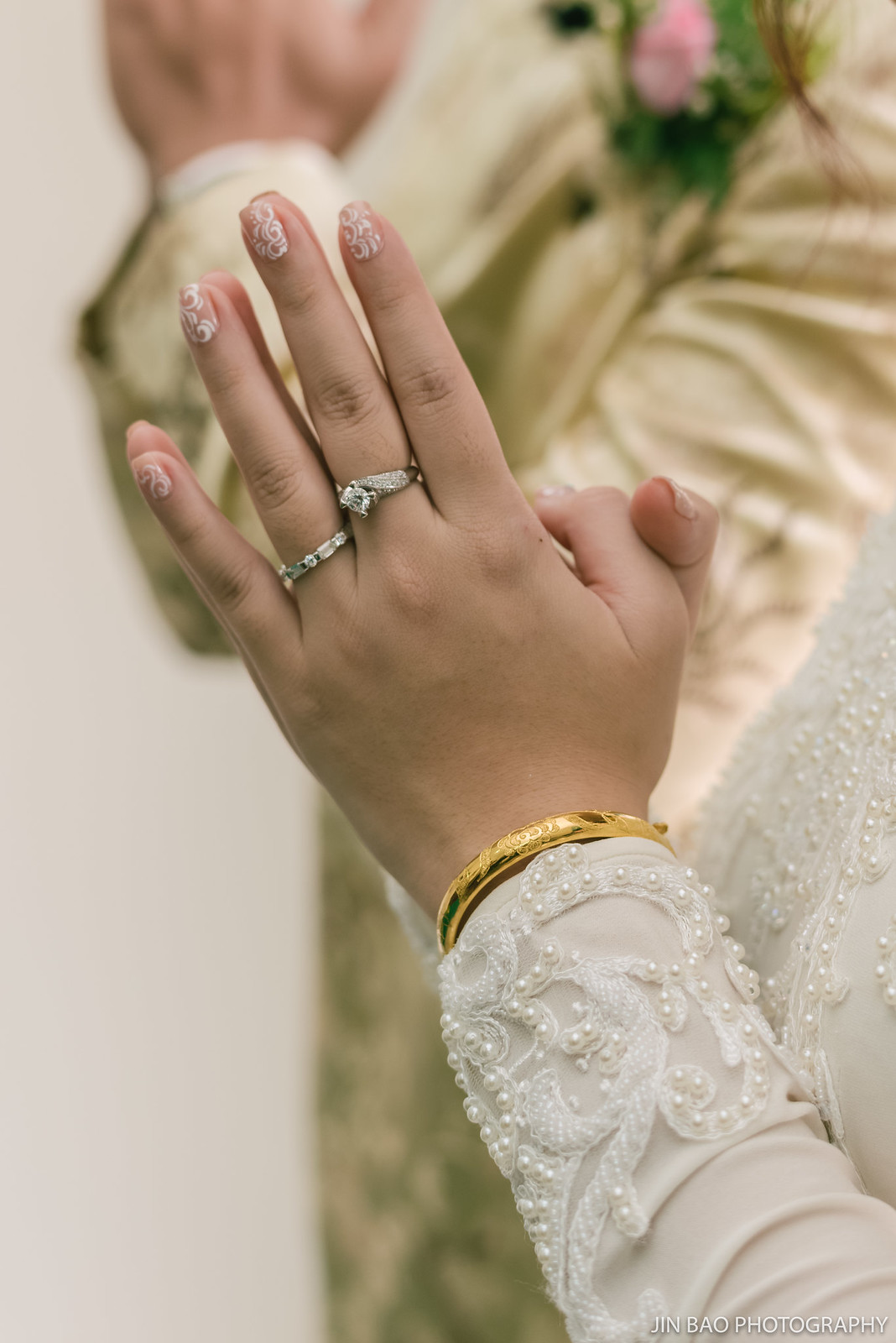The photograph is a close-up of a woman's hands positioned in front of her chest in a praying gesture, with her thumbs crossed over each other. She has rings on her middle and ring fingers, and her nails are painted with a glittery, peach-colored polish displaying wavy patterns. On her left wrist, she wears a golden bracelet. The woman is dressed in what appears to be a white wedding dress adorned with pearls and intricate flower patterns on the chest and sleeves. In the slightly out-of-focus background, a man in a beige suit, also with hands in a praying position, has a pink rose boutonniere on his lapel, suggesting a possible wedding ceremony context.